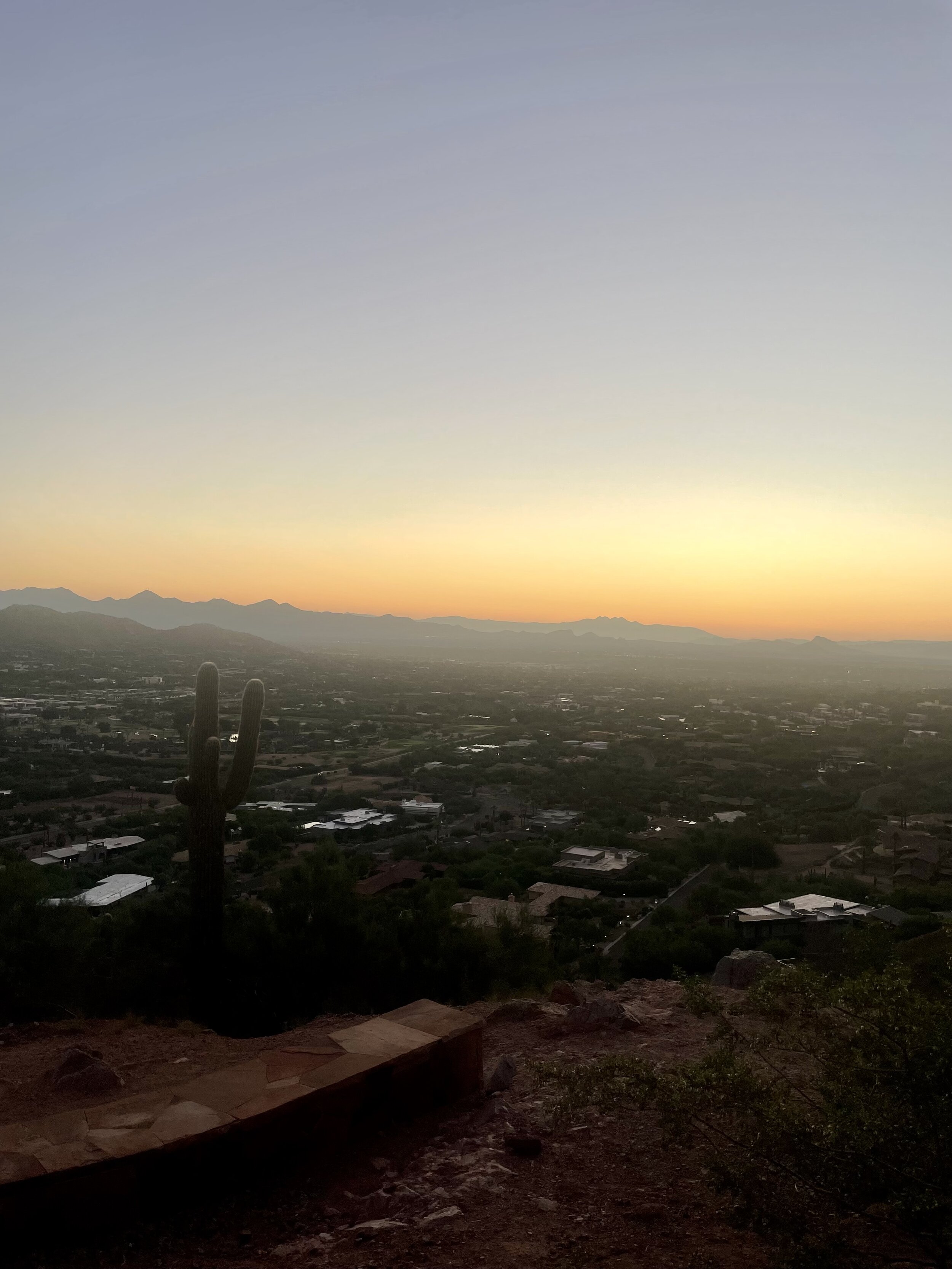The photograph captures a panoramic view from the top of a hill, overlooking a serene town during a sunset or sunrise in a desert region. The foreground features a dirt-covered hilltop with sparse greenery and a notable backless, old-looking bench, accompanied by a visible cactus to the left. Below, a varied landscape of houses is interspersed with trees, suggesting a flat terrain divided by greenery. In the background, a range of mountains or hills adds depth to the scene, and the sky, although described differently, appears mostly clear with a captivating orange hue hinting at the early or late sun. A small stone wall is present on the hill, contributing to the rustic charm of the setting.